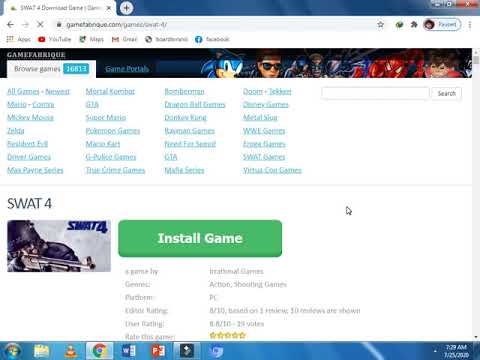This image captures a pixelated screenshot of a Windows XP internet browser window, specifically Internet Explorer, displaying a video game download page. The search bar reveals the URL as "gamefabrique.com/game/SWAT_four/". The title bar features a vibrant collage including iconic characters like Sonic the Hedgehog, The Terminator, Wolverine, Spider-Man, and Sora from Kingdom Hearts.

Below the title bar, there is a navigation tab labeled "Browse Games" with a list of various games displayed in blue text across several columns. The first column lists titles such as "All Games," "Mario," "Mickey Mouse," "Zelda," "Resident Evil," "Driver," "Max Payne," and "Mortal Kombat." The second column includes "Mortal Kombat," "G-16," "Super Mario," "Pokemon Games," "Mario Kart," "G-Police Games," and "True Crime Games." The third column enumerates "Bomberman," "Dragon Ball Games," "Donkey Kong," "Rayman Games," "Need for Speed," "GTA," and "Madden Series." The final column lists "Doom," "Cherry Games," "Metal Slug," "WWE Games," "Apple Games," "SWAT Games," and "Virtua Cop Games."

Prominently displayed in the center of the page is the title "SWAT 4" accompanied by its logo. A large green bar below this reads "Install Game." Directly beneath, in smaller gray text, are sections labeled "Game Specs" and "Game Information," though the specifics are too small to discern.

At the very bottom of the screen, the familiar Windows XP taskbar is visible with several icons: a folder icon, VLC media player icon, Chrome browser icon, WordPad icon, PowerPoint icon, and another browser icon. Additionally, there is an empty Google Chrome icon hinting at a separate, perhaps additional, browser window.